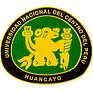This image displays a distinctive circular patch designed to be sewn onto a jacket or shirt. The patch has a detailed, colorful appearance with a prominent yellow, green, and black color scheme. Encircling the patch is a thick black band that contains yellow text, which reads "Universidad Nacional del Centro del Peru" and "Huancayo" at the bottom, indicating its connection to a Peruvian institution. 

Inside the black border, a narrow yellow band frames a green background, which holds a striking central yellow figure. The figure appears to have intricate features: on closer inspection, it looks to some as if it has elements resembling a snake emerging from the left-hand side and a goat possibly holding a staff. To others, the figure might whimsically resemble a monkey with an exaggerated hand seemingly involved in an animated gesture. The combination of symbolic elements and vibrant colors makes this patch a vivid representation associated with its educational origin.